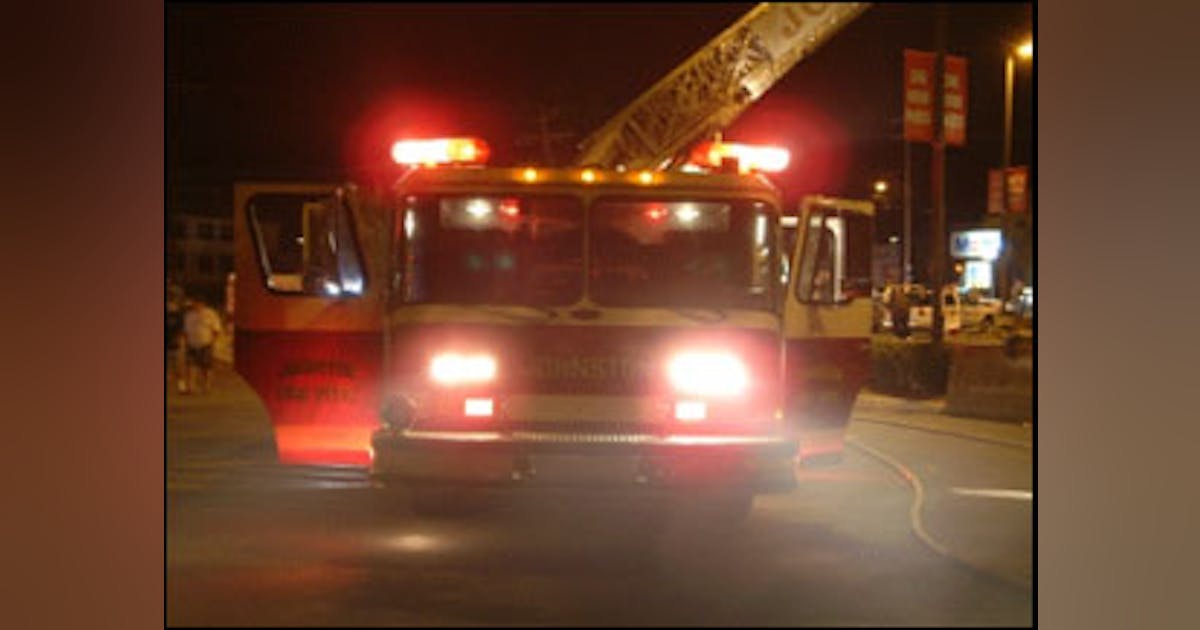In this evening shot, a vintage fire truck from the 1980s or 1990s commands the scene with its vibrant red body and distinctive white trim. The truck is fully illuminated, with red sirens and bright white lights flashing at the front—two large ones and two smaller ones flanking the white grill. The scene appears urban, evidenced by the dark backdrop punctuated with various billboards on the far left and a flagpole adorned with advertisement posters. The ladder, either white or silver, is prominently extended towards an unseen destination, hinting at the urgency of the situation. A fire hose can be seen trailing from the truck's bottom right corner, likely in use at the scene. The overall composition highlights the fire truck's readiness and classic design set against a cityscape under the cloak of night.